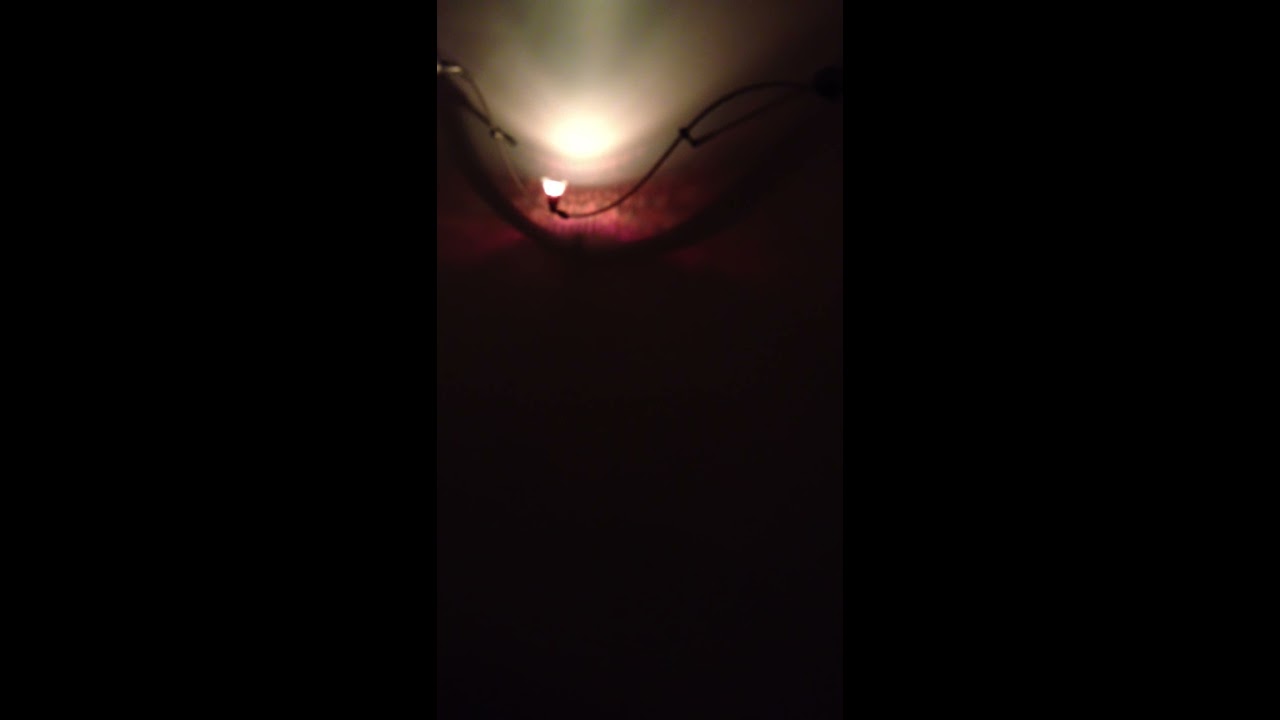The image is a strikingly dark composition dominated primarily by deep shadows. In the upper central portion, a light sconce casts an orb of light and its reflection onto the ceiling, providing the sole source of illumination in the frame. The bottom half of the image is tinged with a subtle yet noticeable red glow. The focal point of the image adopts a 9x16 portrait orientation, bordered on either side by two black vertical rectangles, adding depth and framing the central subject. The image lacks any identifiable people or text and appears somewhat blurry, giving it a cryptic and abstract quality. The overall setup and framing suggest it could have been a cropped capture from a digital platform like Facebook, Twitter, YouTube, or TikTok.